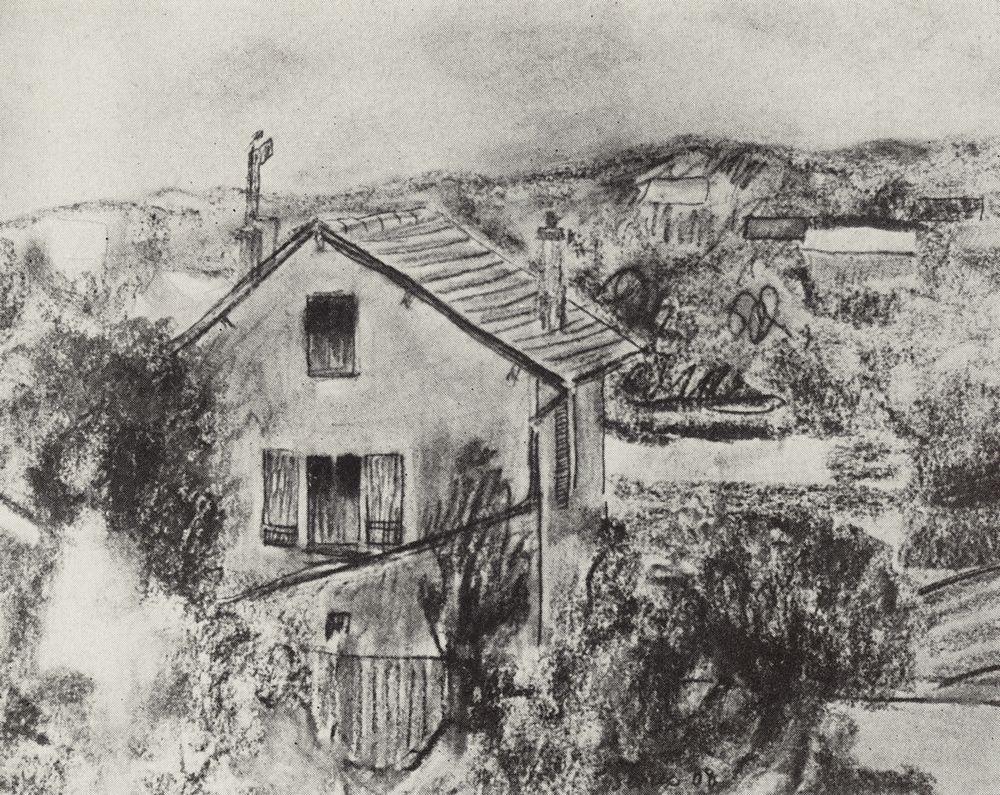This artwork appears to be a charcoal drawing done on white paper, depicting a quiet countryside scene. The primary focus is a stoic, plain house that may resemble a villa, characterized by its wooden shutters and an old-style tile roof. The house stands several stories tall, with a window on each level and features such as a visible chimney and a surrounding fence. In the foreground, there are bushes rich with branches and leaves, adding depth to the image. The landscape includes indications of hills or mountains in the background, with the sky rendered in light charcoal, creating a stormy or foggy atmosphere through smudged and swirling marks. The style of the drawing is rough and sketchy, suggesting quick, gesture-like strokes, with some accidental smearing of the charcoal. Overall, the piece lacks hyper-realistic detail and does not appear to be professionally signed or dated. It measures approximately eight inches by eight inches.